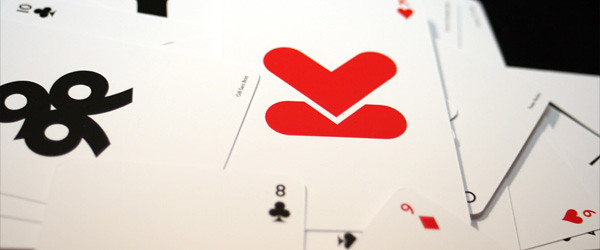This image features a chaotic pile of playing cards with prominently large symbols displayed on their faces. The top card is the King of Hearts, distinguished by its elongated red heart symbol with a base that has a notch, creating a long oval shape. Each card exhibits minimalistic design elements with a single large suit symbol in the center and the card's rank and suit identifier (e.g., "K" and a heart for the King of Hearts) situated in the top corner.

Beneath the King of Hearts, the recognizable symbol for clubs, which appears as three black motifs resembling mirrored and conjoined number nines with an additional nine laid on top, indicates the Ten of Clubs. Among the disorganized stack, visible cards include the Eight of Clubs, the Nine of Diamonds, and the Six of Hearts scattered towards the right side of the image.

The cards rest upon a slightly visible black background, emphasizing their disorderly, overlapping arrangement. Each card's prominent single suit symbol coupled with the rank and suit identifier in the corner provides a stark and clean visual contrast against the haphazard pile.